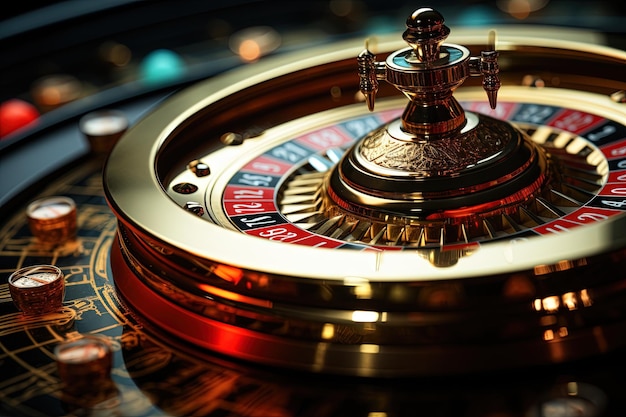The image features a digitally enhanced close-up of a brightly lit roulette table, dominated by an elegant and prominently displayed roulette wheel. The centrally positioned wheel showcases shiny gold rims and a raised gold centerpiece, resembling a hubcap with a decorative piece on top. Surrounding the centerpiece is a circular arrangement of black and red squares, each adorned with white numbers. The glossy gold of the roulette wheel contrasts with the out-of-focus, darker shadows around the rim. The background, devoid of people, consists of colored objects in red, blue, yellow, and orange, adding to the artistic ambiance while maintaining a focus on the shimmering wheel and its intricate details.